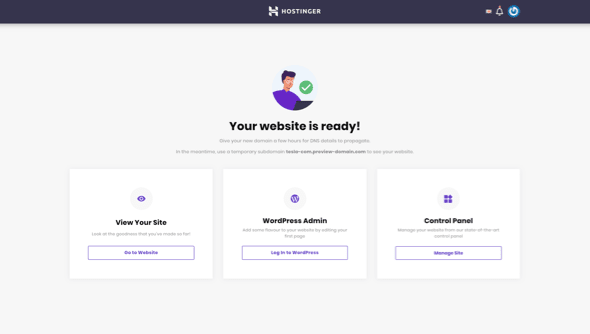This screenshot captures a section of the Hostinger web page. The top of the page features a black border, prominently displaying the Hostinger logo, which consists of a stylized letter "H" followed by the company name "HOSTINGER" in all capital white letters. Towards the upper right corner, there's an icon of a bell with a red indicator at its top, adjacent to a blue circle containing another smaller white circle.

Dominating the center of the page is a small but significant graphic set against a predominantly blank backdrop with some text that is largely out of focus. The key visual element is a circular graphic positioned directly beneath the Hostinger logo. The circle has a blue background, inside of which is an illustration of a woman with dark hair tied back in a bun, wearing glasses and a blue shirt, and looking down at a laptop screen. Embedded within this graphic is a green circle featuring a prominent white checkmark.

Below this image, the largest text on the page reads "Your website is ready" in bold black letters. Further down, obscured by a lack of focus, is some additional text. The bottom part of the screenshot showcases three distinct buttons: the first labeled "View Your Site," the middle one "WordPress Admin," and the rightmost one "Control Panel."